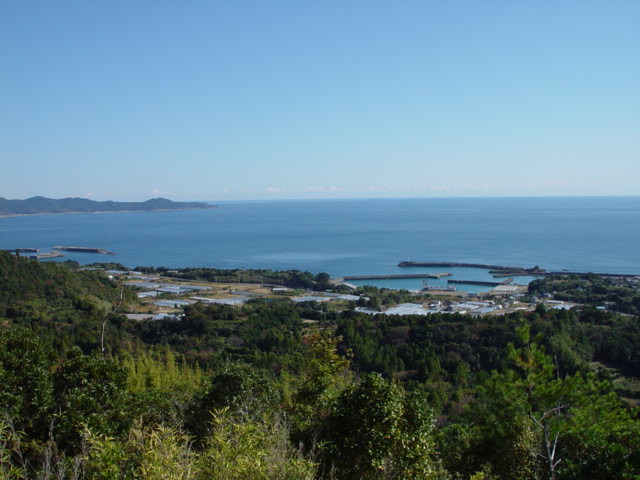This is a detailed, scenic photograph of a seaside view taken from an elevated vantage point, capturing a broad panorama. In the foreground, lush green trees and deep green shrubs frame the scene. To the left, rolling hills sweep down to the shoreline, characterized by a rocky coastline that juts into the blue expanse of water. The midground reveals small, distant buildings and docks, suggesting a sparsely populated area, perhaps a quiet, secluded village. The blue ocean stretches far and wide, contrasting with the crisp, clear blue sky above. This sky fades progressively from a darker hue at the top to a lighter, almost white haze near the horizon. No people or animals are visible in the image, providing an undisturbed, tranquil atmosphere. To the upper left, a particularly prominent rock formation, almost like a small mountain, extends out into the sea. Beyond this, way off in the distance, more faintly visible islands and white clouds dot the horizon, adding depth and intrigue to the overall composition.